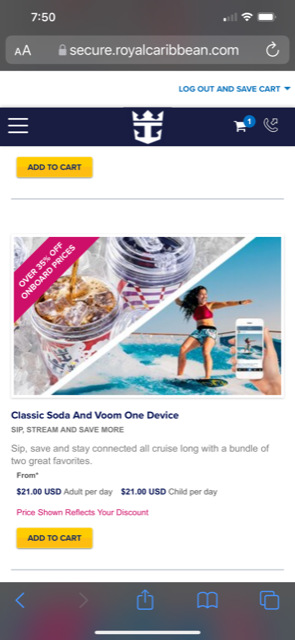**Detailed Descriptive Caption:**

A screenshot from the secure.royalcaribbean.com website shows a promotional offer for onboard services. In the top right corner, options for "Log Out" and "Save Cart" are visible, with a cart icon indicating one item and a call symbol beside a hamburger menu on the left.

The main content includes a vibrant image displaying a woman surfing, captured from below by someone's phone camera. Located above this image are two beverage cups, one with a lid possibly containing coffee and the other with a straw and ice, resembling a soda.

The promotional details boast "Over 35% Off Onboard Prices," offering a classic soda and the "BOOM One Device Ship" package. The tagline encourages travelers to "stream and save more, sip, save and stay connected all cruise long" with two bundled favorites at a price of $21 USD per adult per day and $21 USD per child per day. The displayed price reflects the applied discount. A prominent yellow rectangle button labeled "Add to Cart" is positioned below the offer.